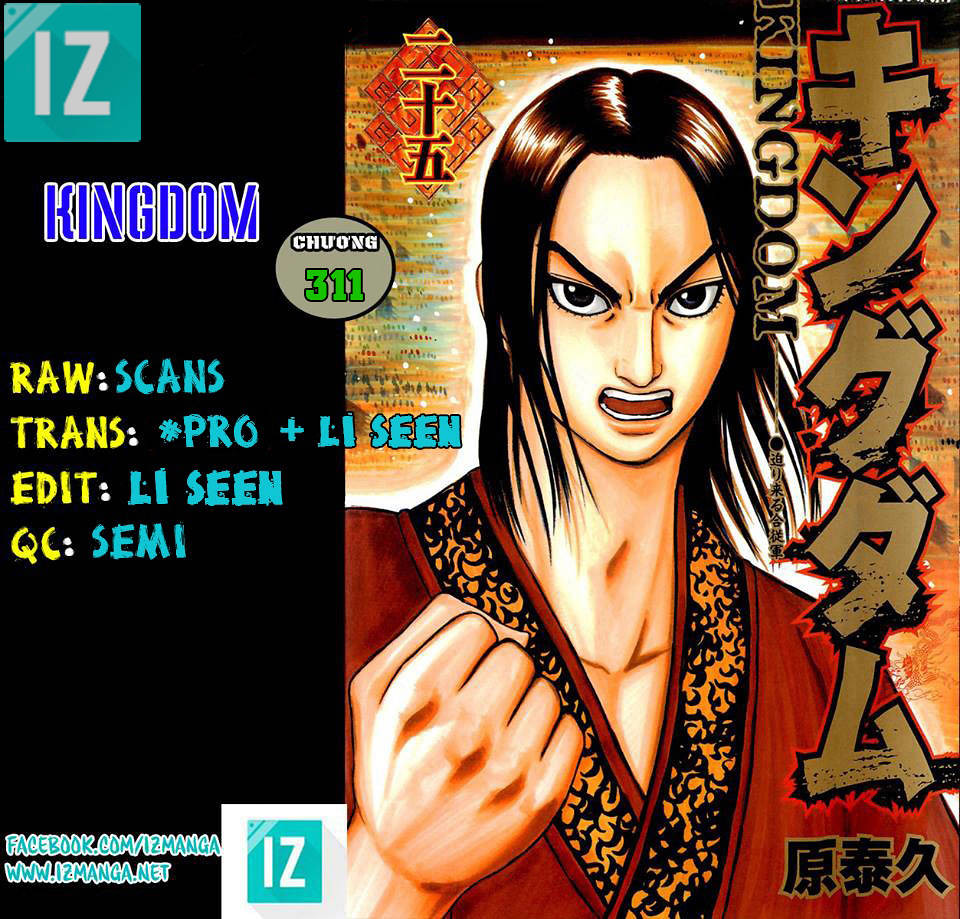The image is a color, square, cartoon or anime-style drawing, likely an advertisement for an Asian manga titled "IZ Kingdom." In the top left corner, "IZ" is written in white within a light green, greenish-bluish square. Below that, in blue letters, is "Kingdom," followed by "Chuong 311." There are further details listed: "RAW: scans," "Trans: Pro Plus L1 Scene," "Edit: L1 Scene," and "QC: Semi."

The right side of the image features a prominently displayed cartoon young male with an angry expression, raising his right fist. He is dressed in a dark red robe with black and gold highlights around the neckline. There is also some foreign writing in a beige-ish brown color. This lower section contains details on the artists involved in the production of the graphic novel, emphasizing the collaborative effort behind "IZ Kingdom."